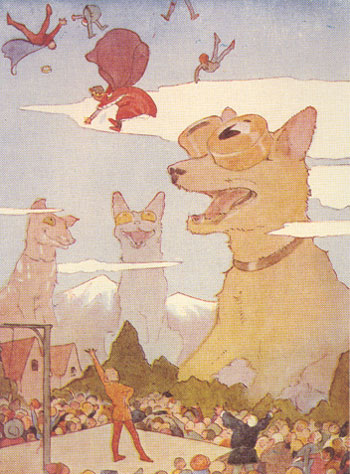This abstract, psychedelic painting features a vibrant scene brimming with surreal elements. At the bottom, a rectangular stage stretches from the bottom center to the bottom left, where a flamboyant performer stands. The performer, clad in an orange suit or jacket and dark orange pants, strikes a dynamic pose with one hand extended and the other on their hip. Surrounding the stage is a lively crowd of cheering spectators. 

Dominating the mid-section of the artwork are three gargantuan dogs, each towering over the landscape and even dwarfing the snow-capped mountain ranges in the background. The dog on the center right is depicted in a vivid yellow, while the other two dogs, positioned to the left, are rendered in light blue and light red hues. These dogs possess hourglass-shaped eyes, adding to their otherworldly appearance.

In the sky above, a clear light blue expanse is dotted with a few clouds, some of which align near the large dogs' heads. Scattered through the sky are five human figures, seemingly falling or suspended in mid-air. Two of these figures, located at the top left, don capes—one red, reminiscent of Superman, and the other blue. Another figure at the top center, mostly cropped out, leaves only his legs visible.

In addition to these elements, there are hints of houses and faint images of more dogs blending into the mountainous backdrop. The entire composition creates a fantastical tableau that challenges reality, merging human forms, giant creatures, and surreal landscapes into one mesmerizing image.